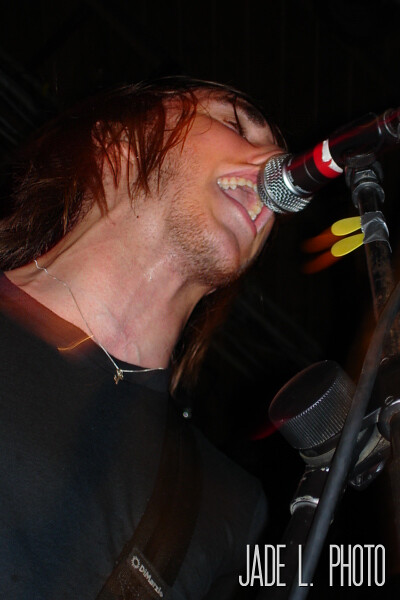The image depicts a close-up shot of a male musician intensely singing into a microphone with a screen mesh head, supported by a stand. Captured from a low angle, the photograph highlights his widened, sweaty neck and face. His mouth is wide open, revealing good teeth, and his eyes appear to be closed as he focuses on his performance. The singer, a white man with long, brown, slightly stringy, sweat-drenched hair, has a stubbly beard. He wears a dark shirt and a thin chain necklace with a small pendant, possibly resembling a key. A guitar strap crosses over his shoulder, although the instrument itself is not visible. The background of the photo is black, emphasizing the bright light shining up from below the stage. The image is signed at the bottom in tall, white letters as "JADE L. PHOTO," indicating the photographer's name, Jade L. Odo. In addition, the strap he's wearing has gray or white writing that reads "Demarxie."